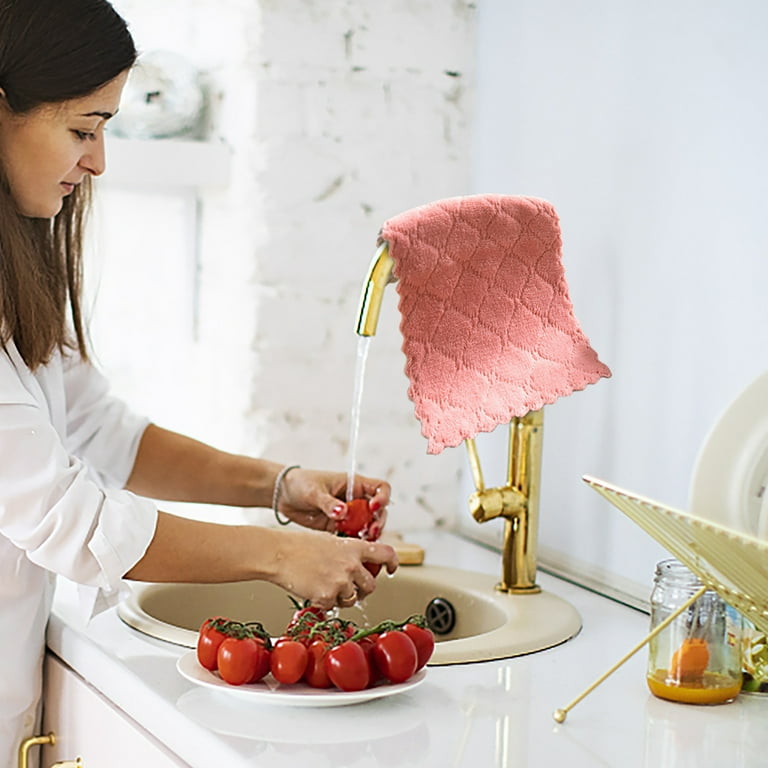The photograph captures a detailed scene of a middle-aged woman with long dark hair, standing at a beige circular sink in her kitchen, washing plum tomatoes. The woman, dressed in a white shirt with sleeves rolled up to her elbows, is positioned to the left side of the image, with both arms extended into the sink, each holding a tomato under the running water. The sink, centered in the image, features a distinctive tall, gold-colored faucet with a peach hand towel draped over its curved top. On the shiny white countertop in front of the sink rests a plate filled with about a dozen plum tomatoes, many still attached to their stems. To the right, a dish rack holds several white plates drying, and next to it, a glass jar containing something orange. The kitchen's sleek design is further highlighted by a white marble background. The overall composition captures a moment of meticulous care and routine in the process of cleaning fresh produce.